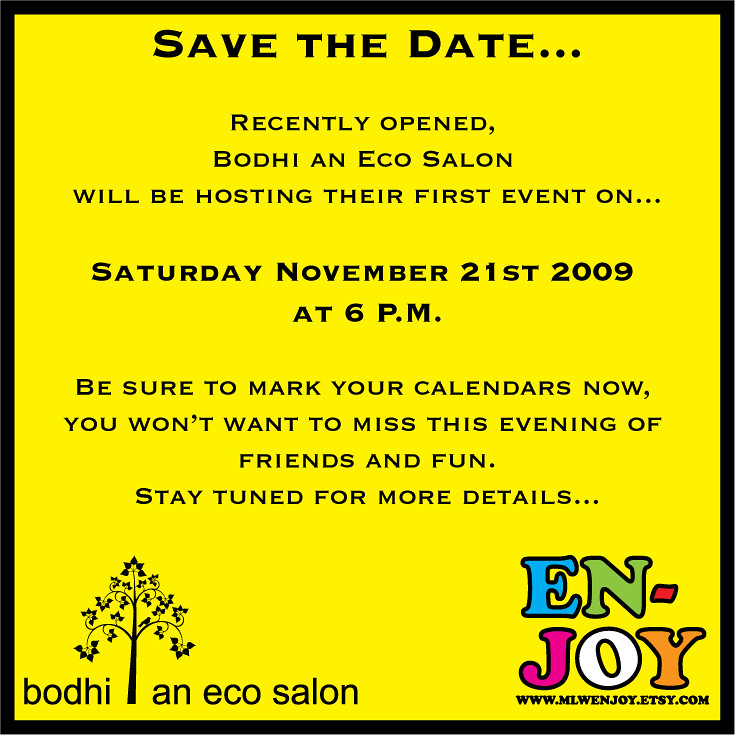This digitally synthesized poster features a prominent yellow background bordered in black. At the top, bold black capital letters announce "SAVE THE DATE." Below, in smaller, unbolded black text, it reads: "Recently Opened, Bode and Eco Salon will be hosting their first event on." Following this, the event details are highlighted in bold black font: "Saturday, November 21st, 2009 at 6 p.m." The next lines, in non-bolded text, urge readers to mark their calendars, promising an unmissable evening of friends and fun, and to stay tuned for more details.

The bottom left-hand corner features a logo consisting of the name "Bode" paired with a cartoon depiction of a tree with flowers as leaves, and the words "Eco Salon" beside it. On the bottom right-hand side, the word "EN-JOY" is displayed in vibrant colors: blue "E," green "N," pink "J," white "O," and orange "Y." Beneath this, in small black font, is the website: www.mlwenjoy.etsy.com.